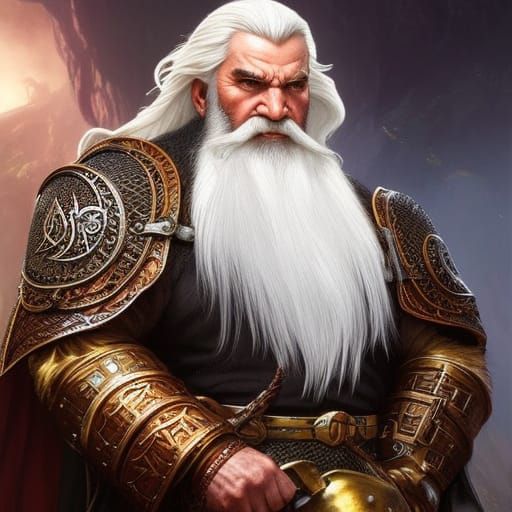In this detailed AI-generated artwork, an elderly man is depicted as a mythical or medieval figure, possibly a dwarf, clad in intricate golden and bronze armor. His striking appearance is marked by long, flowing white hair, a long white mustache, and a wispy beard that extends to his belly button. With a furrowed brow and an expressionless mouth, he gazes off to the right, giving him a stern, contemplative look. His armor includes multi-plated shoulder guards and arm coverings, worn over a black shirt with visible chain mail below a golden belt that features a dagger handle on the left side. The man's hands are mostly bare, except for one hand that is gloved, holding a golden object, possibly a helmet, in front of his waist. The background reveals a dim setting with a dark rock wall or cave-like structure and a hint of a smoky sunset on the left, casting an ethereal glow.